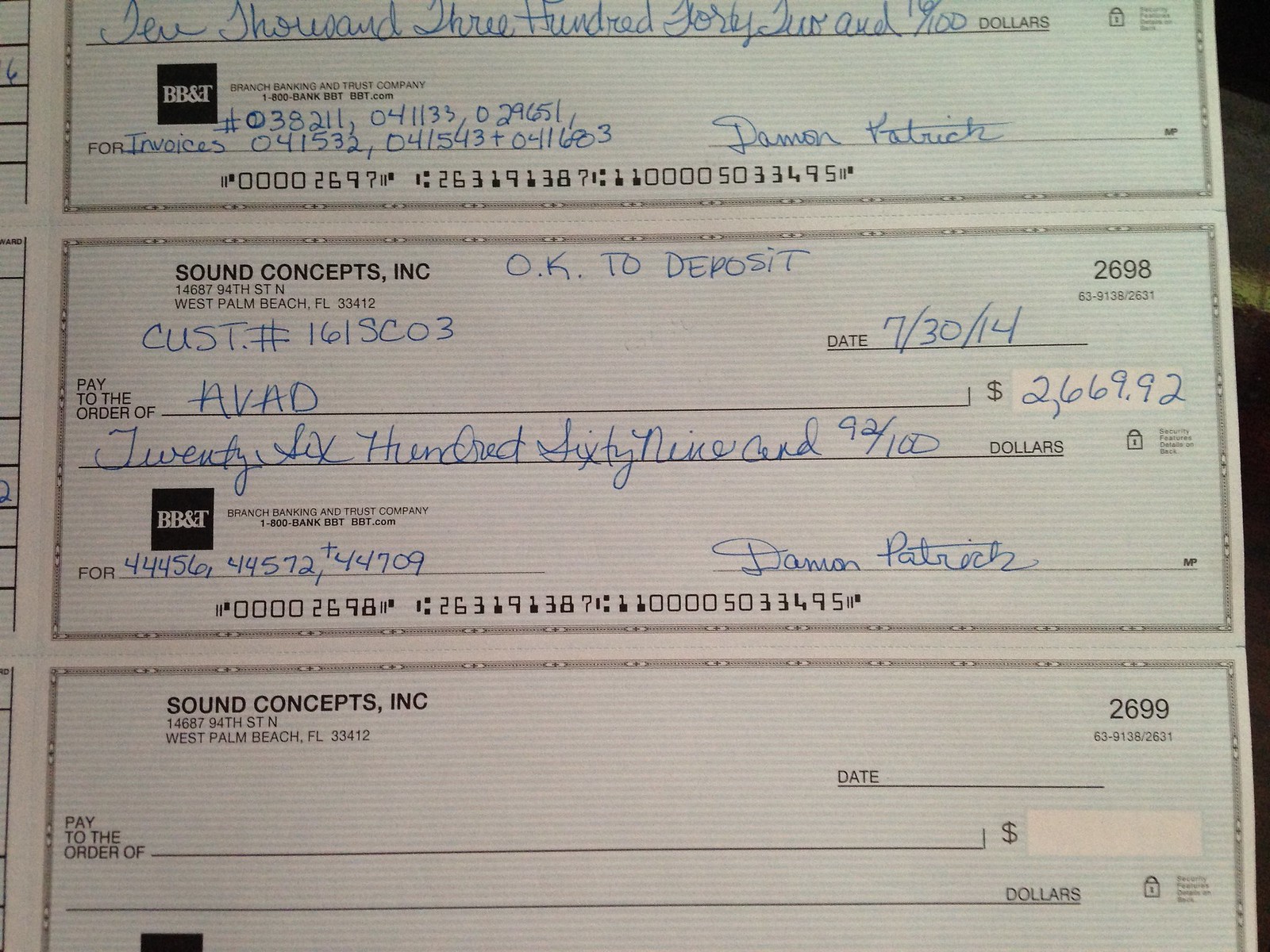This detailed photograph features three bank-issued checks arranged vertically, one above the other, with the top and bottom checks partially out of frame. All checks belong to Sound Concepts, Inc., located at 94th Street North, West Palm Beach, FL 33412, and they share the same routing number: 000-2697-26319-138. The middle check, dated 07-30-14, is fully legible and made out to AVAD for $2,669.92. This check includes multiple invoice numbers and is duly signed. The top check, partially visible, is written for $10,342 in blue ink, but crucial details such as the payee's name are obscured. The bottom check remains unused, displaying no information except its check number, 2699, and is entirely blank. The image highlights the middle check, with the majority of the information clearly visible and emphasizing the company's routine financial transactions.